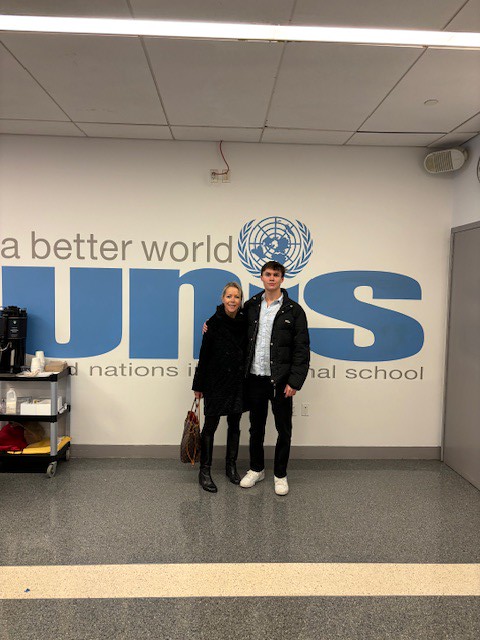In the photograph, a tall Caucasian man and a Caucasian woman stand in front of a large sign that partially reads "A Better World" along with the United Nations symbol. The sign appears to reference the United Nations, possibly suggesting "United Nations National School," though the full text is not visible. The man, positioned on the right, has his arm around the woman on the left. Both are dressed for winter; he wears a winter coat and sneakers, while she sports a black jacket, black boots, and carries a black bag. They are inside what appears to be an office building with yellowish walls adorned with blue text. A coffee tray leans against the wall to their left, and there is a cart with items further to the left. The gray floor features a yellow stripe, and to the right, the room includes doors and a speaker mounted in the upper right corner. The ceiling is white, enhancing the indoor lighting.